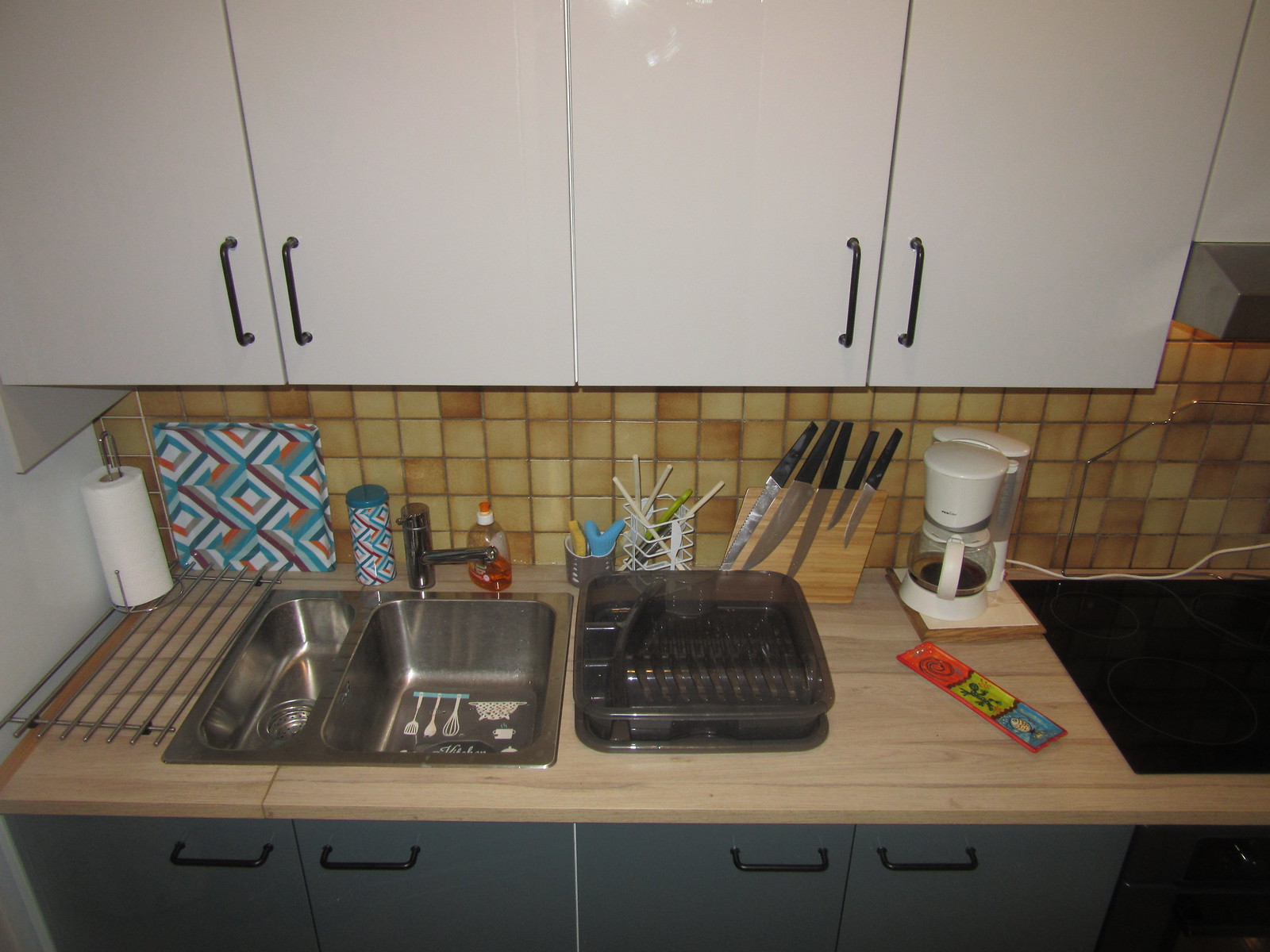The photograph showcases a pristine kitchen area adorned with white Formica cupboards, each equipped with sleek black handles. At the center of the layout is a dual-section silver sink accompanied by a matching silver faucet. Adjacent to the sink, a practical drying rack stands ready for dishes. An upright roll of paper towels is conveniently placed nearby, facilitating quick clean-ups. A white coffee machine with an extended cord claims its spot on the countertop, indicative of daily use. Also occupying space on the counter is a black electric stovetop, streamlined into the kitchen's design. Inside the sink, various silverware pieces are visible, highlighting signs of recent use. Adding a vibrant touch, a hand-painted spoon rest with intricate red, yellow, and blue designs sits on the countertop. The countertops themselves are a light-colored wood, possibly crafted from bamboo, offering a warm and natural aesthetic to the kitchen's overall ambiance.